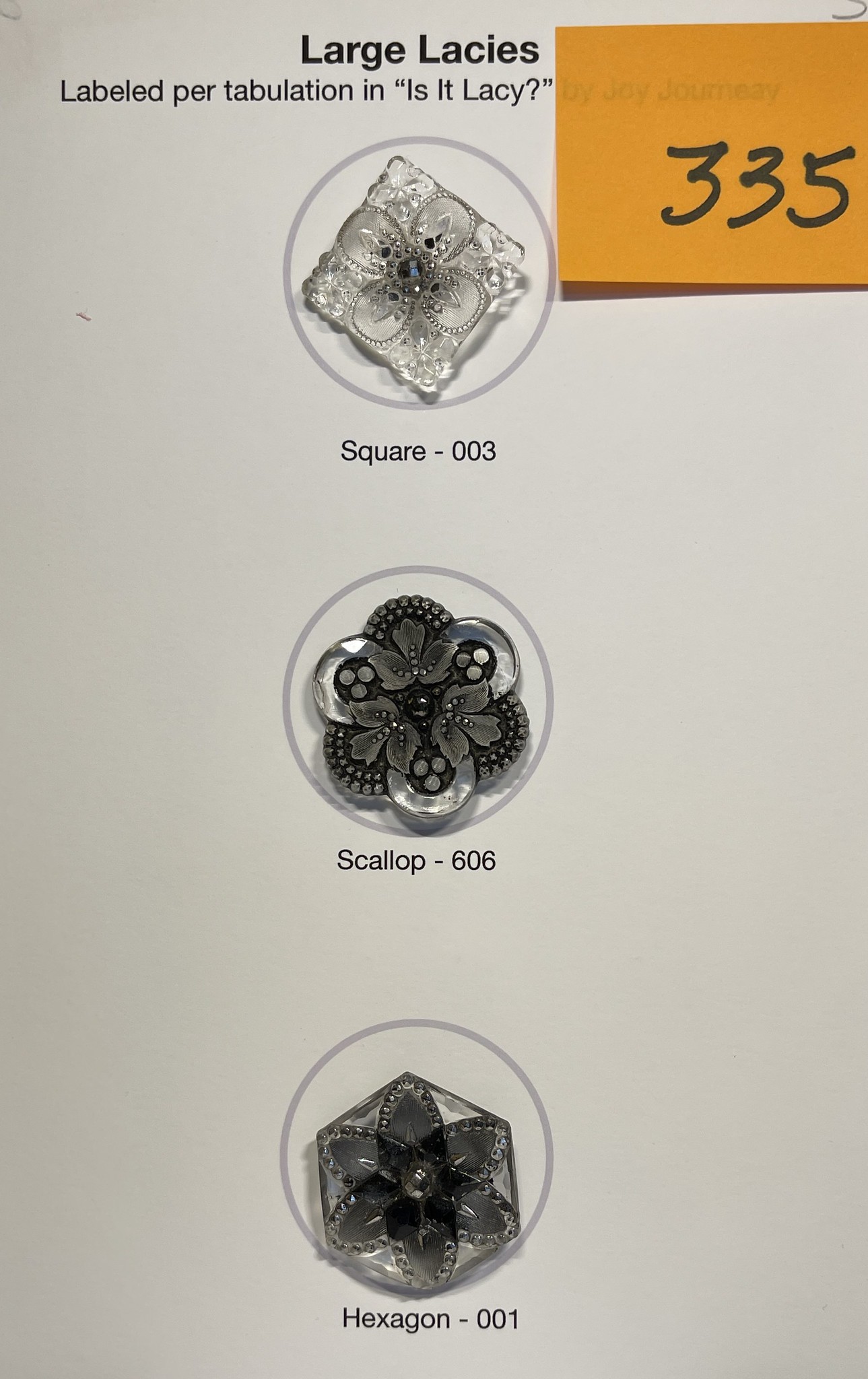The image features a plain gray background adorned with various labels and elements. At the very top, the text "Large Laces" is prominently displayed, and beneath it, the phrase "Labeled per tabulation in 'Is it Lacy?'" appears in quotation marks. In the upper right corner, an orange sticky note with the number "335" is attached. Below the text are three gray circles, each containing intricate designs, resembling pieces of jewelry. The first circle hosts a diamond-shaped, transparent design with three inner circles, appearing like a square rotated into a diamond, suggestive of a piece of delicate jewelry. The second circle, labeled "Scallop 606," features a flower design with leaves and flower buds, crafted from gray metal. The third circle, denoted as "Hexagon 001," displays a six-sided geometric pattern with an internal flower design, all in black. Together, these elements create a cohesive and detailed visual composition on the backdrop.